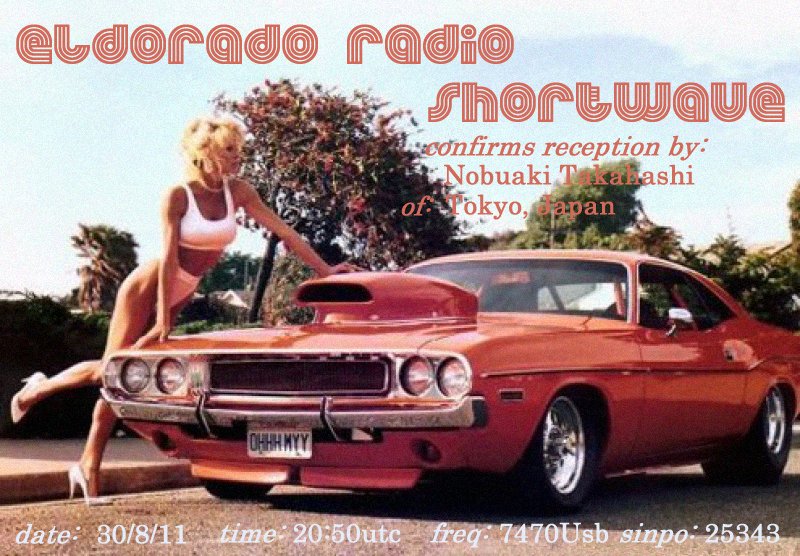The vintage image features an orange muscle car prominently positioned in the center, its large chrome wheels and thick dragster rear tires giving it a powerful stance. The car has a hood scoop and a white license plate on the front that reads "OH MY." Leaning against the vehicle is an attractive woman with blonde hair, dressed in a white sports bra paired with light pink bikini bottoms, and white high heels. She is positioned on the right-hand side of the car. In the background, the scene is framed by lush green trees, a clear blue sky, and scattered white clouds. The image, which has a retro aesthetic, appears to be an advertisement. Overlaying the image, in red text at the top, it reads "Eldorado Radio shortwave confirms reception by Nobiaki Takahashi of Tokyo, Japan." At the bottom of the image, it states in white text: "Date: 3-8-11, Time: 20:50 UTC, Frequency: 7470 USB, SIMPO: 25343."